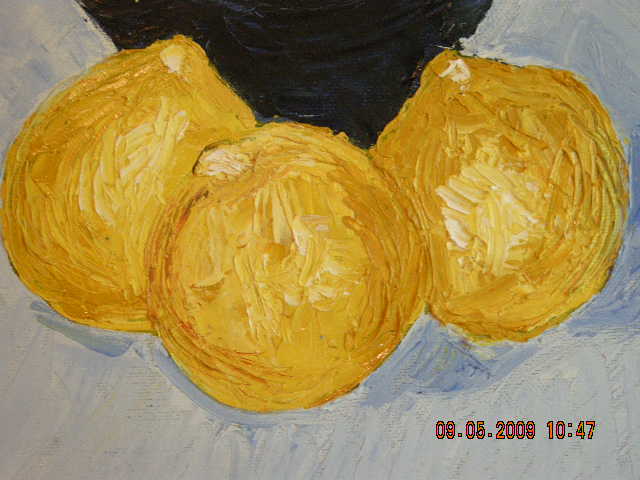This image is a detailed, close-up photograph of a painting, identifiable by visible paint strokes and the texture of the applied paint. At the center of the composition are three yellow, almost orange-hued fruits arranged closely together in a slightly overlapping formation. The fruits resemble melons, coconuts, or possibly lemons, with two displaying a lemon-like point at their tops, while the middle one lacks this feature. Behind the fruits, a black, triangular shape partially obscured by the fruits adds contrast to the predominantly white, subtly blue-toned background. In the bottom right-hand corner, a red digital timestamp reads "09.05.2009 10:47," indicating the photograph's capture date and time.